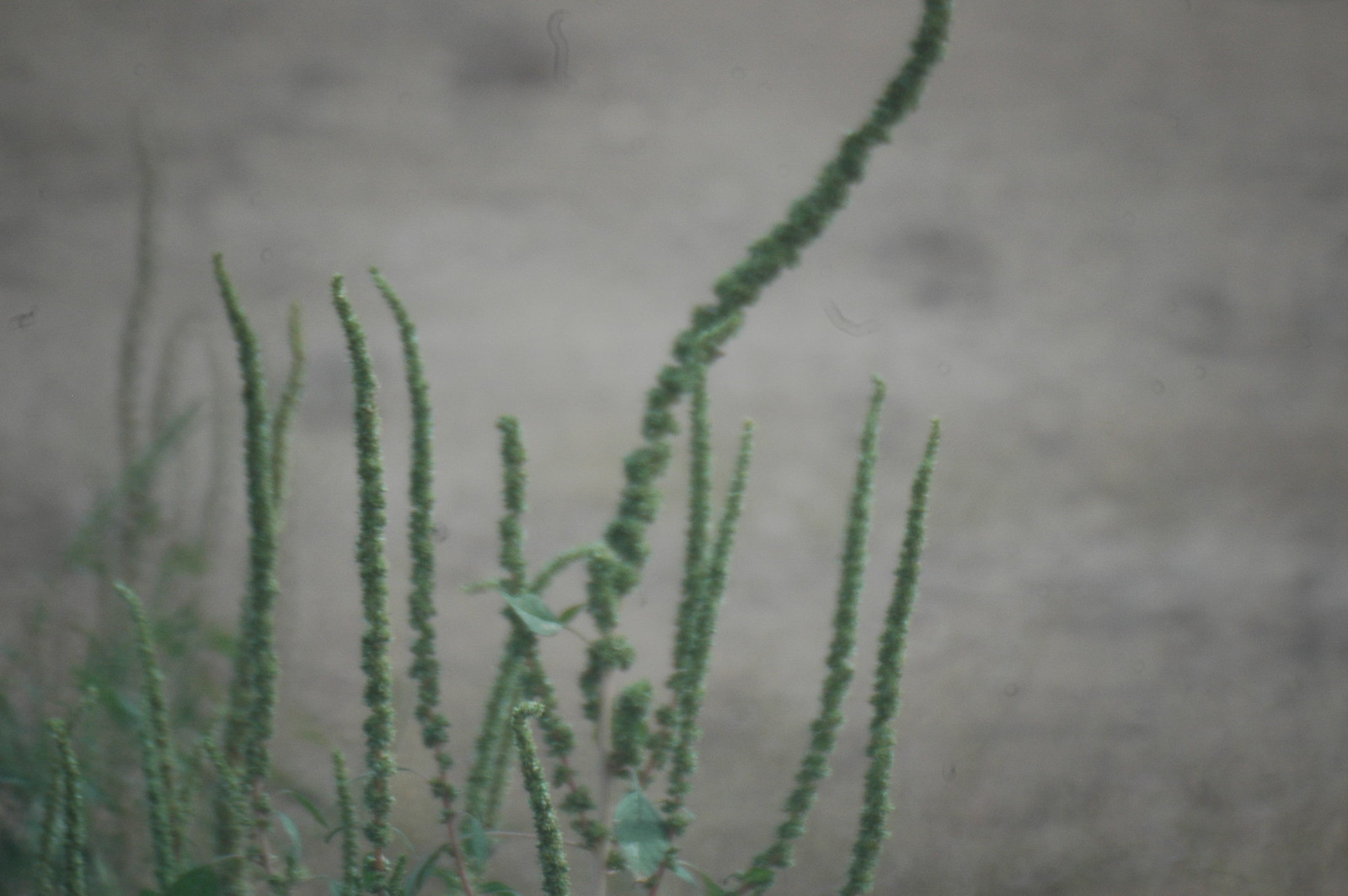This blurred photograph captures an intriguing, green plant characterized by its long, brown stems and sparse, stick-like leaves. The plant, which dominates the bottom left and middle portion of the image, features unique, rounded green structures that resemble flower pods. One prominent stem extends from the bottom center of the frame, growing upwards and extending out of the image's top edge, emphasizing its height. The background is an indistinct gray, with varying darker gray shades, providing a muted contrast to the plant's organic forms. The overall image has a dull color palette and lacks clarity, with the camera positioned closer to the ground, making the green plant the focal point against the blurred, nondescript backdrop.